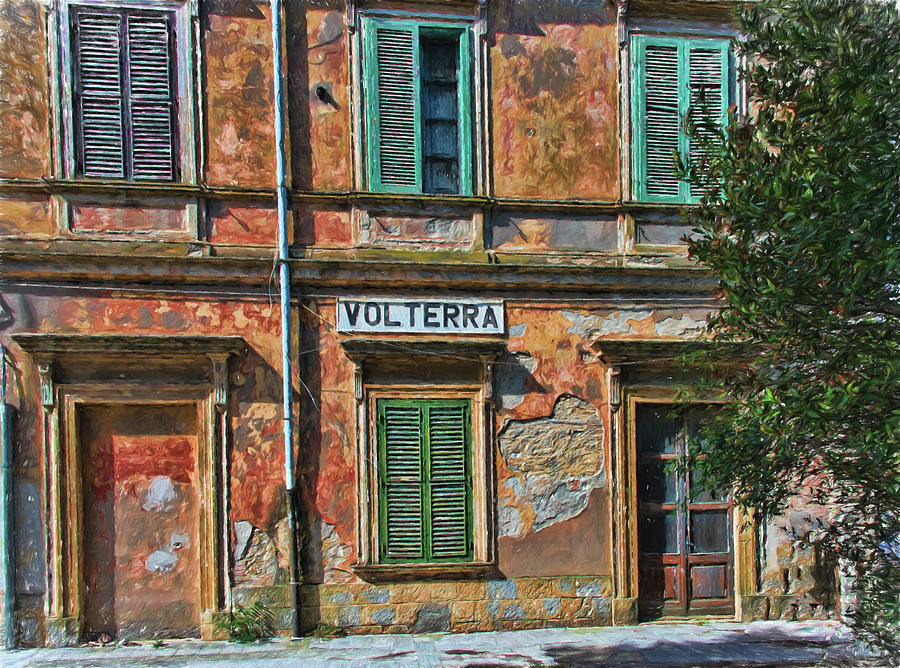This image captures an old, dilapidated building with distinctive architecture. The structure is primarily brown and orange with marks of weathering and age. It features a variety of colorful shutters on the windows; on the second floor, there are purple and blue shutters, and two turquoise shutters on the right side. The building is labeled with a sign that spells out "Volterra" in clear white letters. There are two doors on the bottom floor. One door, made mostly of wood, has six small glass panels, while the other door is boarded shut. The walls of the building are cracked and display a mix of gray, red, dark gray, and orange hues. Additionally, there's a green bush or tree growing along the right side of the building, and a utility line runs in front of the structure. The overall scene hints at abandonment and the passage of time.